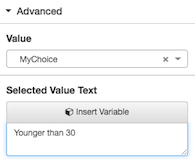The screenshot depicts a low-quality, blurry interface of a menu, either from a website or an application. The background is vividly white, making the text and interface elements stand out, despite the blurriness. 

At the top-left corner, the word "Advanced" appears in a slightly blurred black font, accompanied by a small arrow pointing diagonally down to the left. Below this label, a slender grey line serves as a separator.

Underneath this grey line, the word "Value" is displayed in black font. Directly below, a small black rectangle contains the text "My Choice," followed by a small 'X' icon in the top-right corner and a downward-pointing arrow indicating a drop-down menu.

Another grey line follows, distinguishing a new section of the menu. This section begins with the phrase "Selected Value Text" in black font. Beneath it, a grey rectangle features an icon of a cube next to the text "Insert Variable."

Adjacent to this icon-text pair, there is a white drop-down menu outlined in light blue. The menu currently displays the text "Younger than 30" in black font, a phrase that carries ageist connotations.